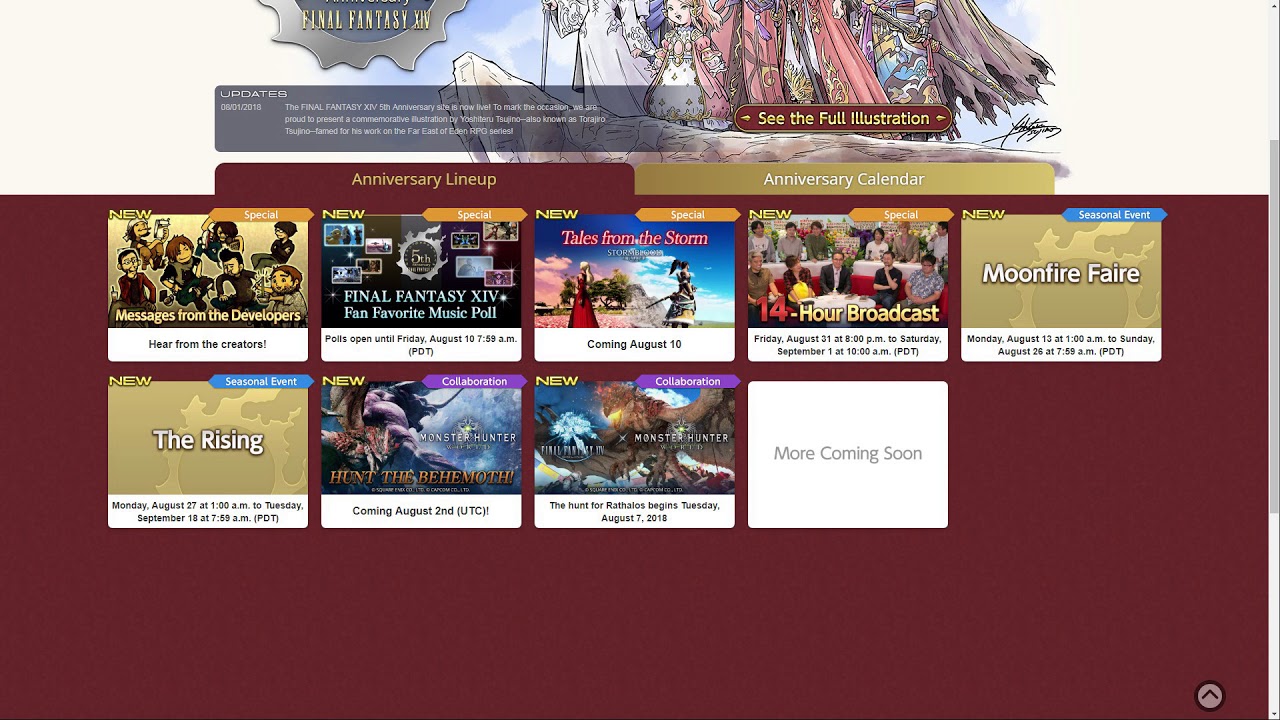Screenshot of an e-commerce website dedicated to Final Fantasy XIV. The header, partially obscured, indicates the top portion either being cut off or scrolled. On the left side, part of a crest with "Final Fantasy XIV" below it is visible. To the right, graphic artwork showcases characters in long, flowing, tattered robes and wielding swords, with a young child prominently positioned in the front, all standing on a rock overlooking a cliff.

A scrolling field on the left is labeled "Updates for Final Fantasy," along with a clickable option to view the full illustration. Below this section, a maroon field with two tabs is present: an "Anniversary Lineup" tab and a gold "Anniversary Calendar" tab. The content under these tabs includes a variety of options such as messages from developers, creator insights, open polls, a music poll, "Tales from the Storm," a 14-hour broadcast likely resembling a live podcast, and events like Moonfire Fair, The Rising, and Hunt of the Behemoths with Monster Hunter. This site appears to provide comprehensive updates and options related to Final Fantasy XIV.